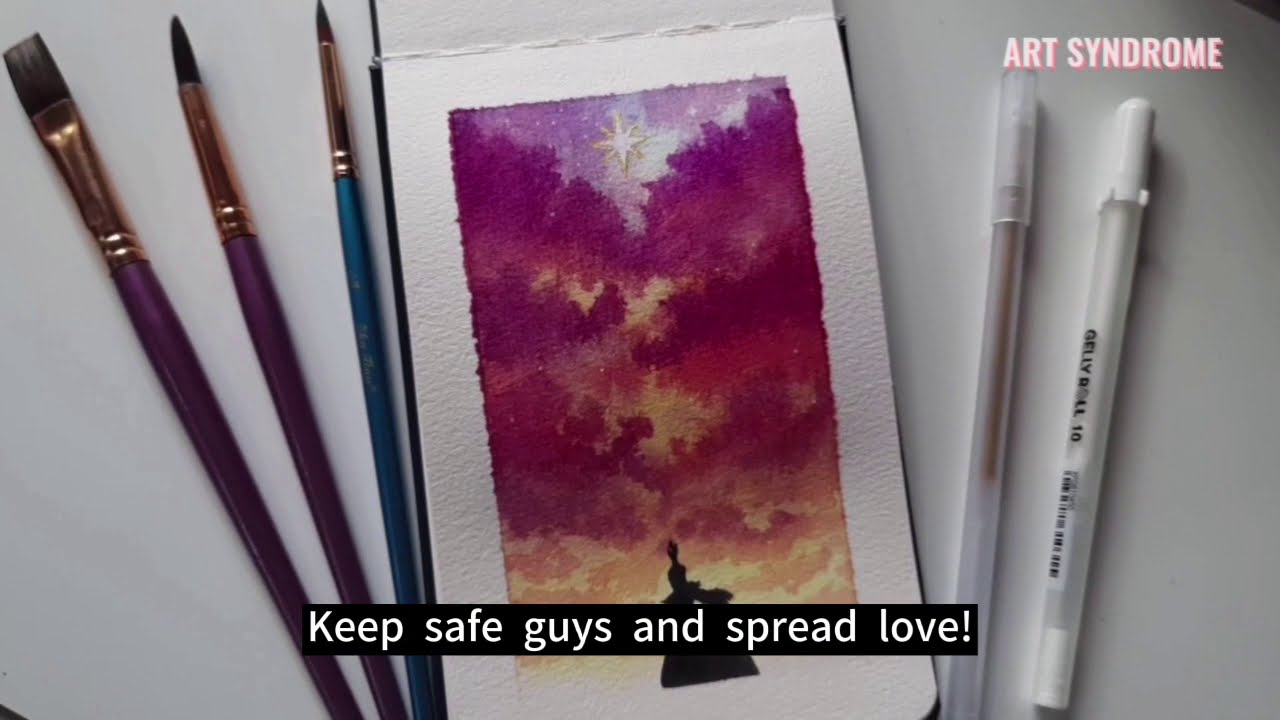The image features a painting on what appears to be thick, textured cardstock, centrally placed on a white surface that resembles a counter or table. The painting, which has a rectangular white border, depicts a vibrant sky with a star at the top. The sky transitions through rich colors, including shades of purple, red, orange, and yellow, resembling a sunset or layered clouds. Below the sky, there is a black rectangle with white text saying, "Keep safe guys and spread love." The background of this text gives a YouTube caption-like appearance. 

To the left of the canvas, there are four paintbrushes arranged in a row, with the largest on the far left and progressively narrower ones toward the center. The two largest brushes have purple handles with gold and black tips, while the third has a blue and gold handle. There seems to be a bit of ambiguity about the fourth item, whether it's another brush or just the edge of the painting. 

On the right side of the canvas, there are two pens with clear bases, one with a clear lid and the other with a white lid. Above these pens, the words "Art Syndrome" are written in light pink, all-caps letters.